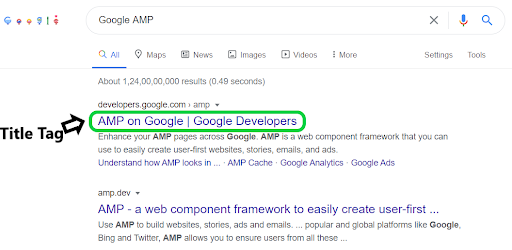Here's a detailed and cleaned-up caption for the image:

---

The screenshot captures a Google search results page where the query "Google AMP" has been entered. The "All" tab is selected, displaying a comprehensive list of results rather than filtering by Maps, News, Images, Videos, or other categories. 

At the top of the results, the first link directs users to the AMP section within the Google Developers website, highlighted by a caret mark. The text snippet under this link reads: "AMP on Google - Google Developers. Enhance your AMP pages across Google. AMP is a web component framework that you can use to easily create user-first websites, stories, emails, and ads." There is also a clickable link suggesting further exploration into how AMP integrates with AMP Cache, Google Analytics, and Google Ads.

The second search result points to the AMP.dev website. The accompanying text describes AMP similarly: "AMP, a web component framework to easily create user-first websites, stories, ads, and emails. Use AMP to build on popular and global platforms, including Google and Twitter. AMP ensures optimal user experience across these platforms."

---